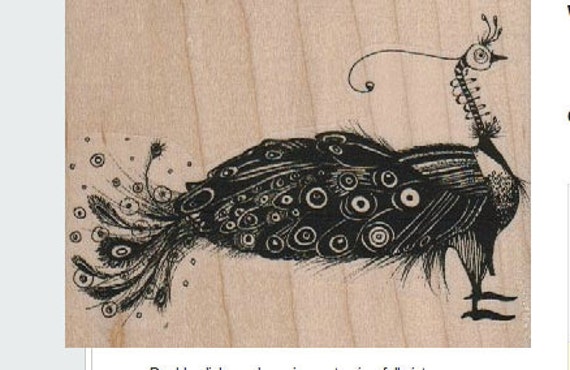The image depicts a detailed, artistic drawing of a peacock rendered in black on a light-colored, wood-grain background, resembling pine. The drawing is oriented in landscape mode, with the peacock facing towards the right. The peacock is shown in a side view with wings and tail feathers closed, emphasizing intricate designs and circular patterns within the black feathers. It features a distinctive thin, long neck adorned with a spiral line, topped with three prominent head feathers. The facial details include a large eye and a triangular nose. The peacock's two legs and feet are also depicted clearly. The style and medium suggest the artwork could be burnt, stamped, or sketched onto the wood, giving it a unique, tattoo-like appearance.